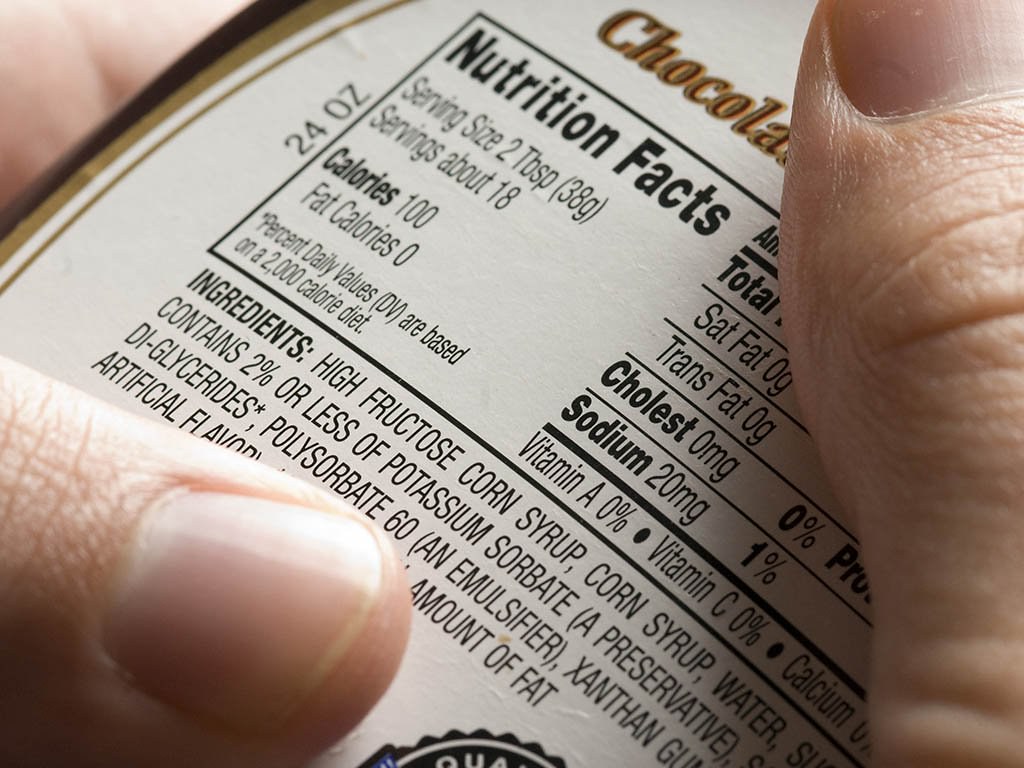This image depicts a close-up of a white Caucasian individual's hands holding a bottle, likely of a chocolate-flavored product. Only their thumb and another finger are visible, partially obscuring the label. The label is white with some gold and brown detailing and features the nutritional information. Key details include "chocolate" prominently written in gold, and the bottle holds 24 ounces. The nutrition facts reveal each serving size is 2 tablespoons (38 grams), with about 18 servings per container, each providing 100 calories and 0 fat calories. Despite being high in sugar, with high fructose corn syrup, corn syrup, and water as primary ingredients, there are no substantial nutritional benefits, as it contains 0% Vitamin A, Vitamin C, and Calcium. The label lists other ingredients like potassium sorbate (a preservative), diglycerides, polysorbate 60 (an emulsifier), xanthan gum, and artificial flavoring. This detailed scrutiny suggests the product might be a type of chocolate-flavored syrup or spread.